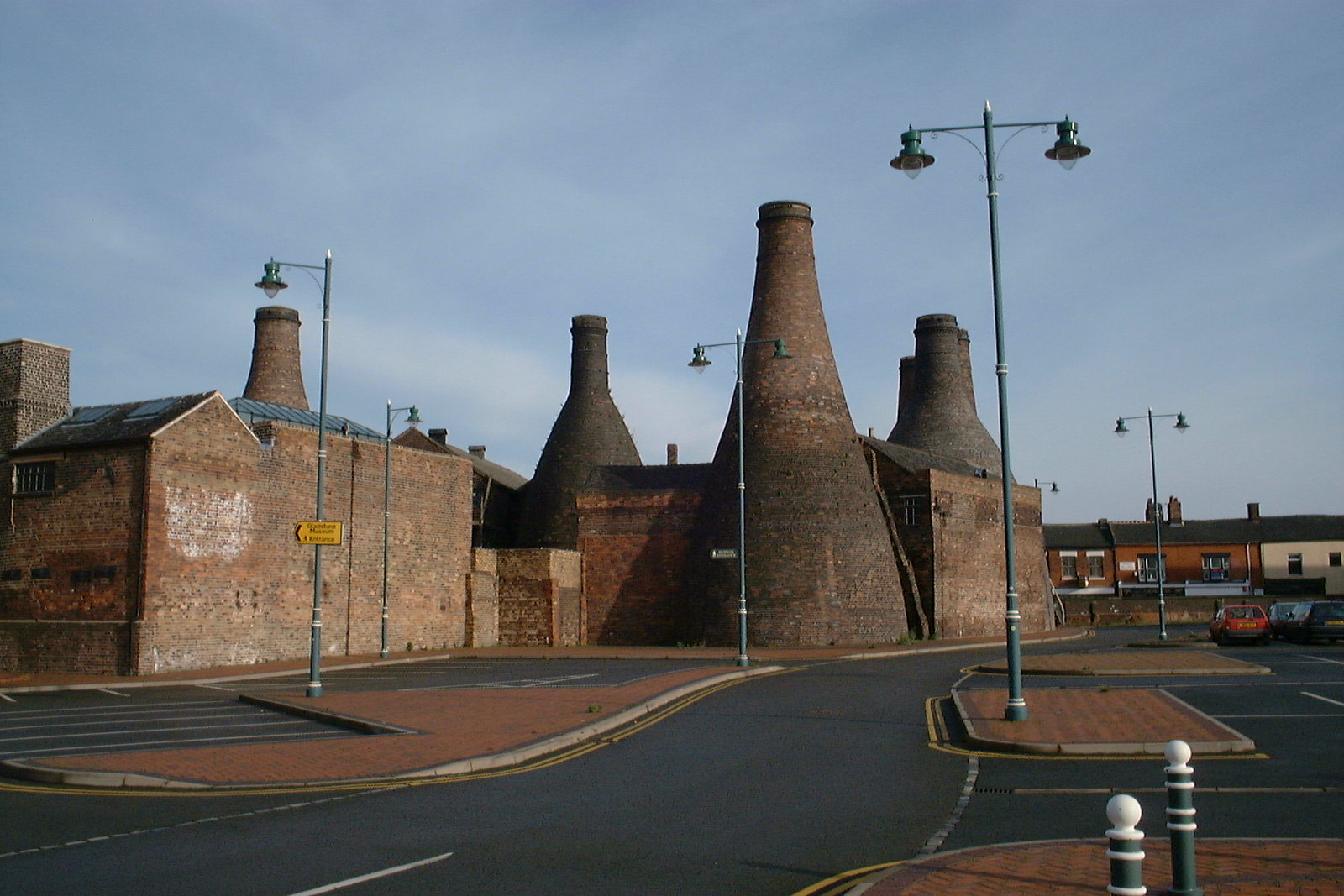The outdoor image reveals a hazy sky backdrop with an ensemble of brick and white houses, reminiscent of townhouse styles, located in the far distance. Dominating the foreground is a sprawling parking lot punctuated by several brick islands, each adorned with tall green streetlights. Two cars are visible, situated towards the distant edge of the lot. Central to the scene is a distinctive brick structure, characterized by four towering smokestacks that are conical in shape, broad at the base and narrowing towards the top, each about twice the height of the brick building they sprout from. Additional brick buildings surround this structure, adding to the industrial atmosphere. The presence of worn yellow signs and license plates suggests a European setting, further implied by the architecture and signage reminiscent of regions like England. The vantage point captures brick islands with light poles, a roadway, and a turn lane, emphasizing the structured layout of this possibly historical industrial site, perhaps once used for kilning or burning, given the design of the smokestacks.